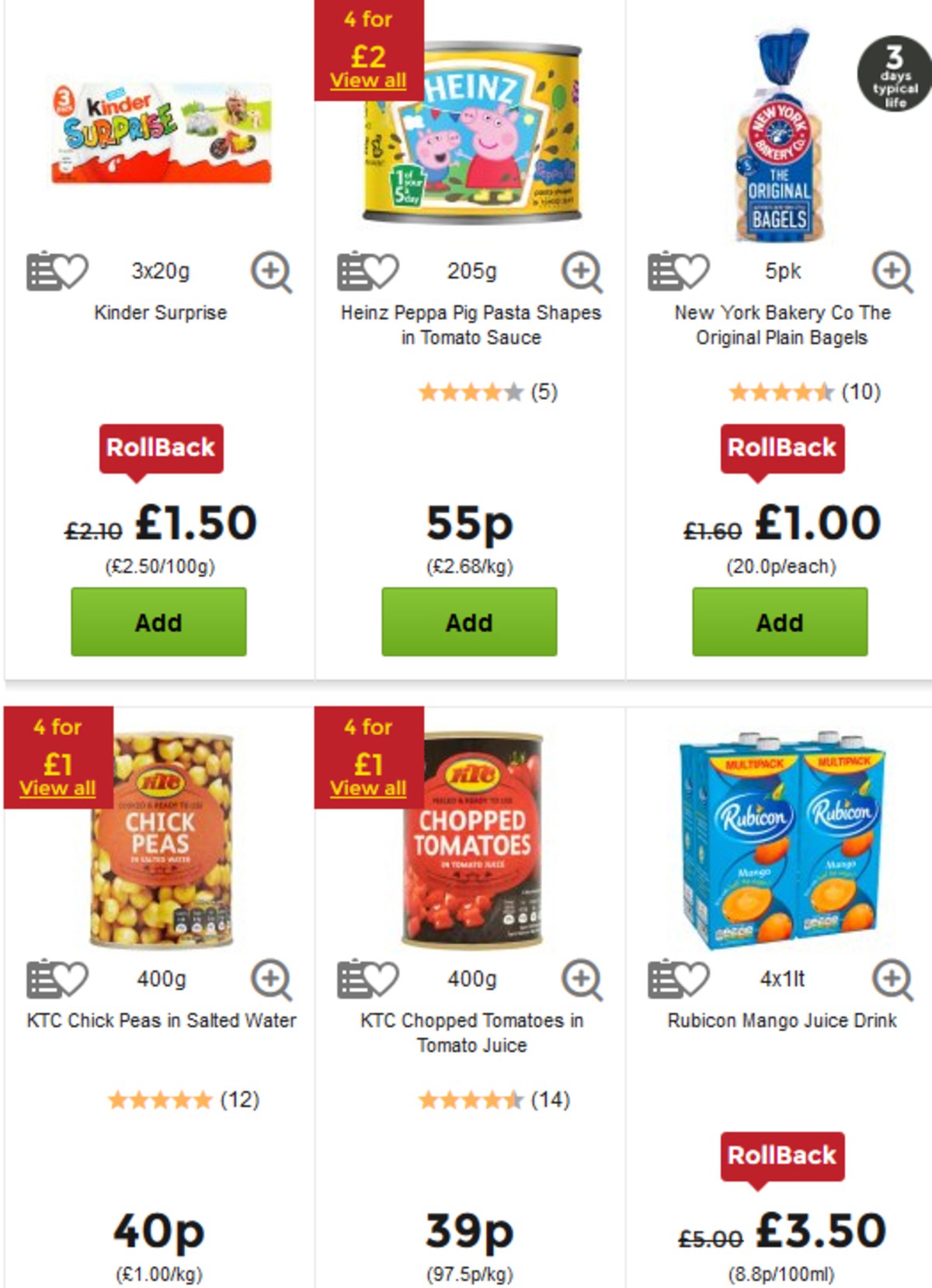The image features a printout of a website displaying a variety of food items arranged in three columns, each column containing two items. Although some information is blurred, the details are as follows:

- In the first column, the top item is Kinder Surprise, marked as a rollback item in red, priced at $1.50, accompanied by a green "add" button.
- Directly below, Heinz Peppa Pig Pasta Shapes in tomato sauce are displayed, having received four stars based on five reviews, priced at 55p, and also featuring a green "add" button.

- The second column starts with New York Bakery's original plain bagels, listed with a red rollback button, priced at $1.00, and a green "add" button.
- Below it is KTC Chickpeas in salted water, boasting five stars from 12 reviews and priced at 40p.

- The third column's top item is KTC Chopped Tomatoes in tomato sauce, rated four and a half stars out of 14 reviews and priced at 39p.
- Beneath it, Rubicon Mango Juice Drink is displayed as a rollback item in red, priced at $3.50.

Each food item is accompanied by a clear price indication and a green button for easy addition to the shopping cart.